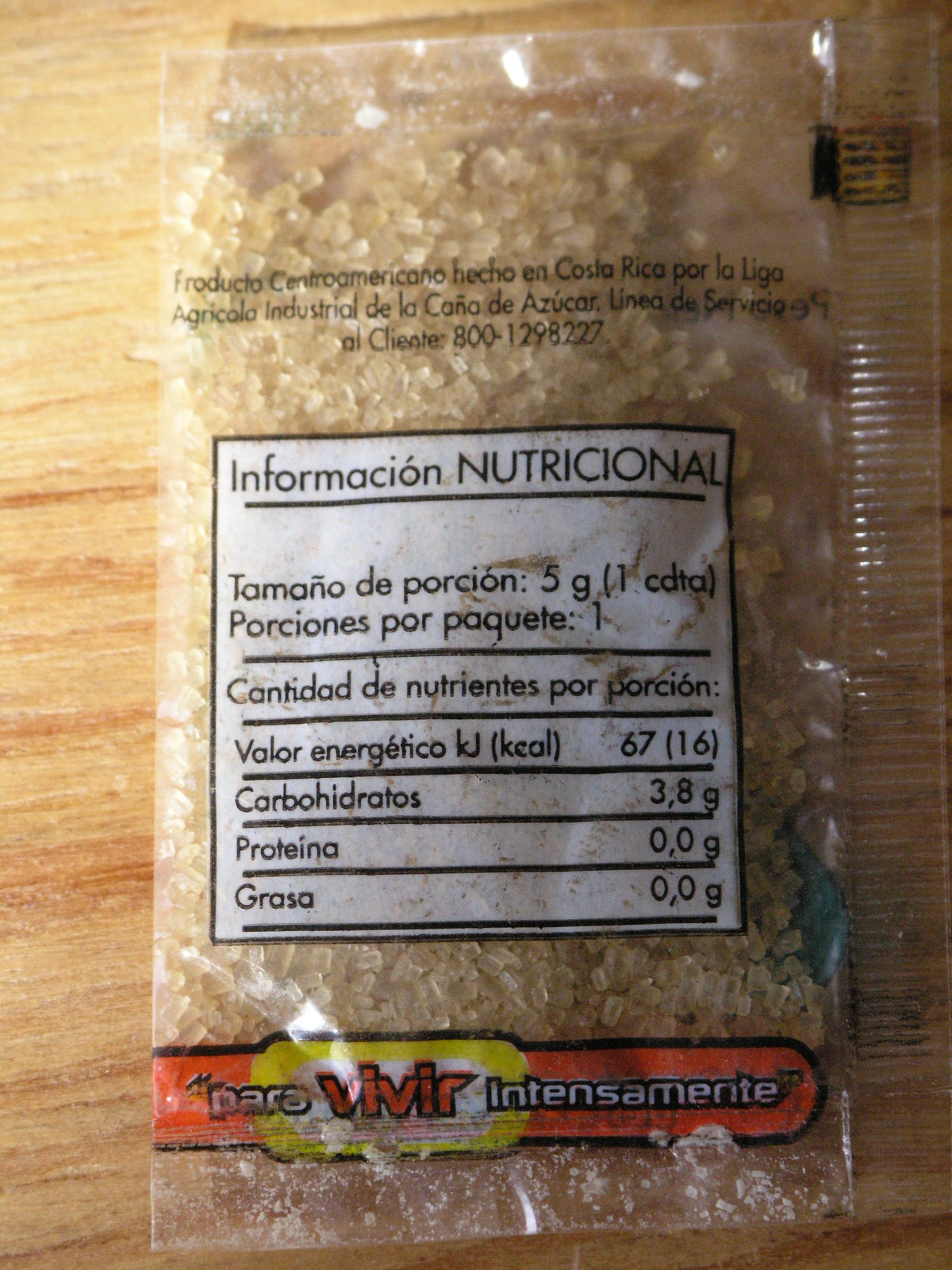A clear plastic bag labeled with the brand name "Freducto Centroamericano" contains oatmeal. The bag is adorned with various inscriptions: "Hecho en Costa Rica," signifying its country of origin, "Por La Liga Agricola Industrial de la Caña de Azúcar," indicating that it is produced by the Agricultural Industrial League of the Sugar Cane, and a product line designation "Linea De Cereal." The packaging prominently displays the product's slogan, "El Cleaner Cheater," along with a contact phone number, 800-129-8227. 

Nutritional information is clearly provided, stating: each serving size is 5 grams, with one serving per packet. The nutritional content per serving is detailed as follows: Energy Value: 67 KJ, Carbohydrates: 3.8 grams, Protein: 0.0 grams, Fat: 0.0 grams. Additionally, the packaging includes the phrase "Para Vivir Intensamente," suggesting a lifestyle-oriented marketing appeal.